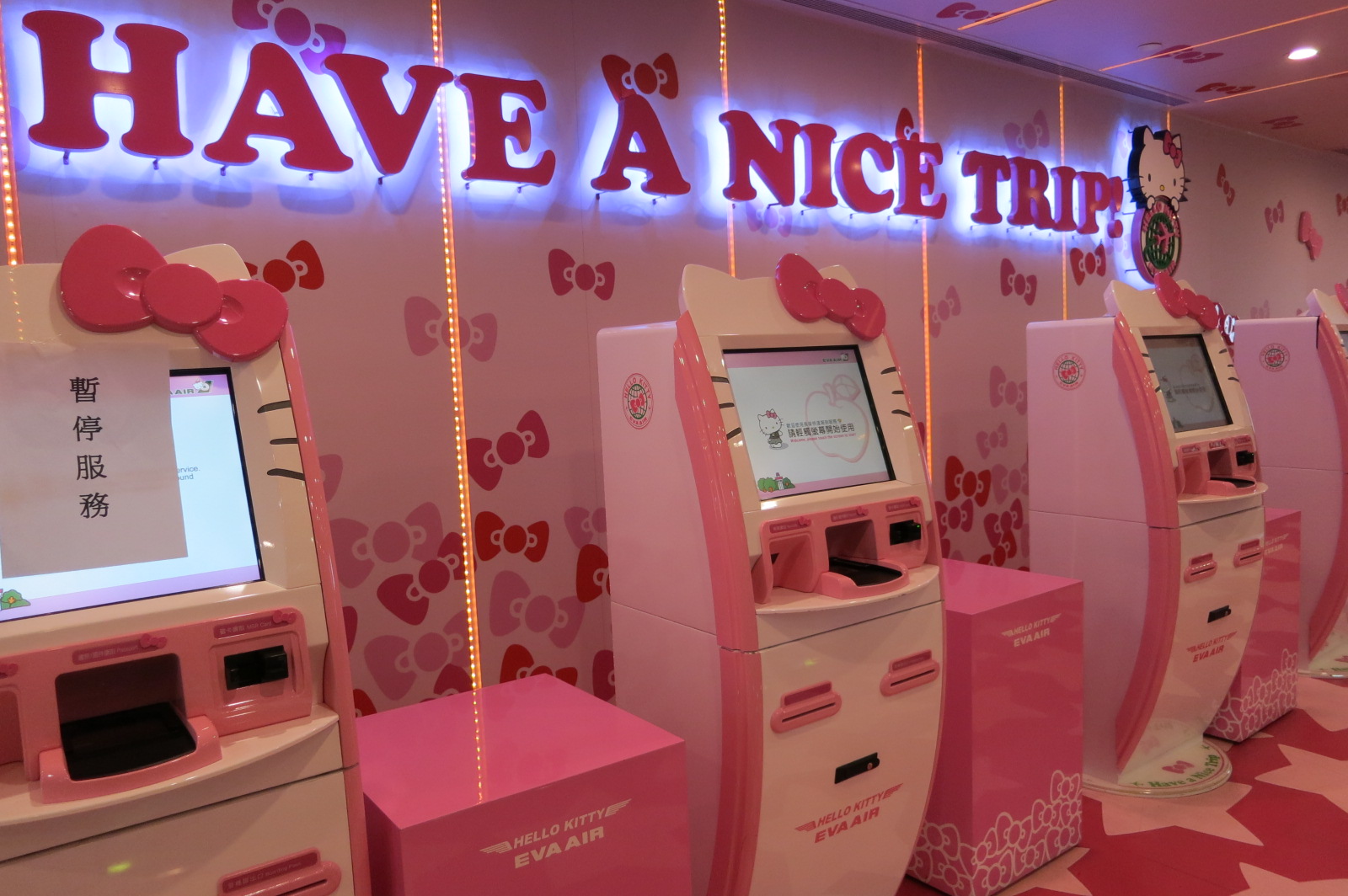The indoor photograph captures a vibrant Hello Kitty-themed setting predominantly adorned in shades of pink and white. Four curved, self-service kiosks, used perhaps for buying airline tickets, stand prominently in the image. Each kiosk is decorated with pink bowls and features the iconic Hello Kitty design; pink bows adorn the kiosks and the wall behind. One kiosk has a screen displaying Hello Kitty with Asian writing. A prominent sign reads "Have a nice trip," accompanied by a large Hello Kitty logo featuring the famed white cat with a pink bow on her right ear. The background wall is white and festooned with seven pink bow ties. Between the kiosks are pink and white boxes labeled "Hello Kitty EVA Air." The flooring continues the pink and white theme. Notably, the leftmost kiosk has a white paper with Chinese or Japanese characters, suggesting it might be out of order. The setting is devoid of people, focusing solely on the cheerful and vibrant Hello Kitty décor.